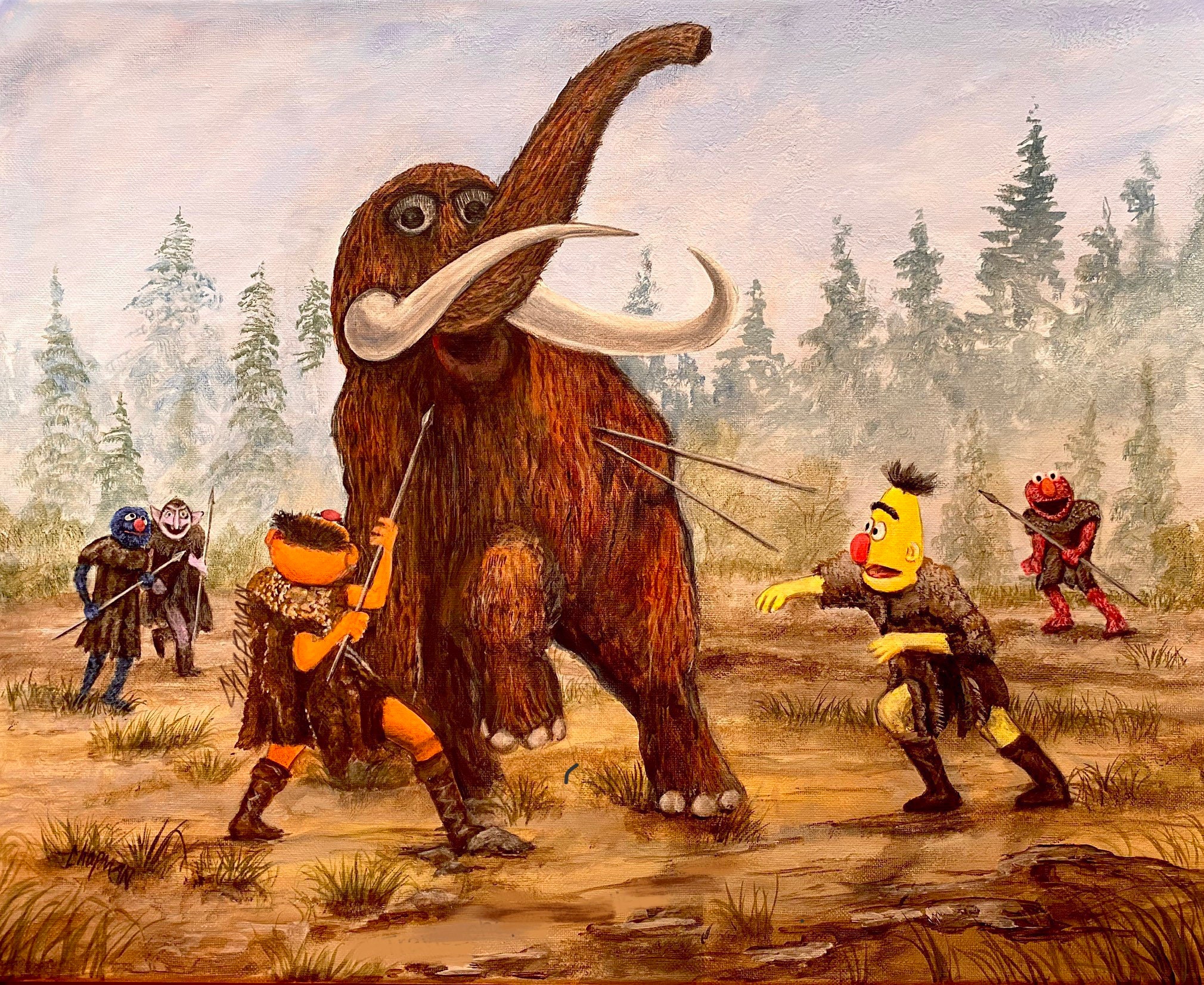A detailed and cleaned-up caption combining the key elements from the three descriptions:

In this horizontally aligned, rectangular canvas art piece, iconic Sesame Street characters are depicted in an unusual, warrior-like scenario. Positioned on a dirt ground with scattered patches of grass, Bert and Ernie are dressed in brown tunics and tall leather boots, resembling ancient warriors or Vikings. Bert (on the left) and Ernie (on the right) are engaged in a dramatic confrontation with a large, friendly-looking woolly mammoth, thought to be a caricature of Snuffleupagus. The mammoth, with its smiling demeanor, large eyes, and long trunk reaching to the upper right, is portrayed with raised arms and two spears embedded in its side. Ernie, holding a spear, aims it towards the mammoth's mouth, suggesting an imminent attack. Surrounding them in the background are additional Sesame Street characters: Elmo, Cookie Monster, The Count, and Oscar—all observing the scene. The backdrop features tall evergreen trees and a cloudy, foggy sky, enhancing the surreal and whimsical nature of the artwork. This vivid and imaginative scene is meticulously painted, showcasing a blend of familiar childhood icons in a fantastical and unexpected context.